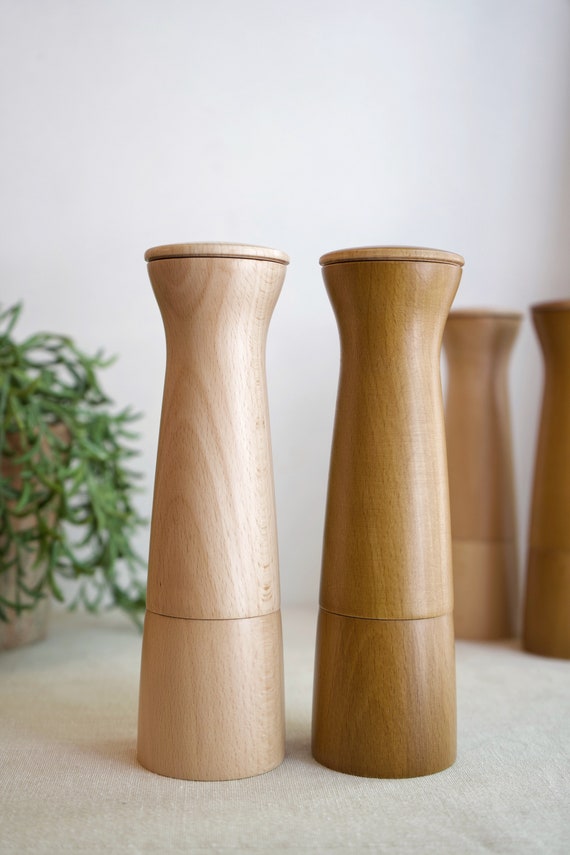In this image, the foreground prominently features a pair of handcrafted wooden salt and pepper grinders. The grinder on the left is a lighter tan color, while the one on the right is a rich, deeper brown. These grinders are positioned on a white or beige fabric, possibly a tablecloth, which adds a soft, homely touch to the scene. Each grinder has a noticeable groove around a quarter of the way up, indicating the part where the mechanism possibly turns or fits together, and they both have removable caps at the top. Complementing the scene, a small green potted plant sits to the left of the grinders. In the background, slightly out of focus, another pair of similar grinders can be seen, echoing the aesthetic of the foreground items. The setting appears to be a cozy living room, suggesting a warm and inviting domestic environment.